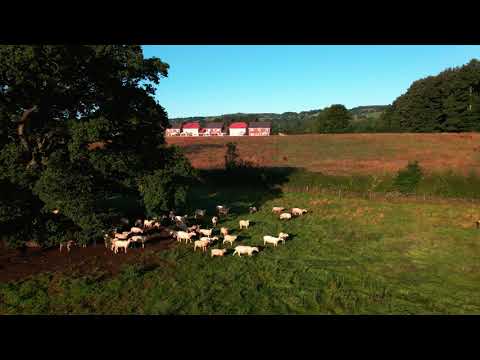This horizontally aligned rectangular photograph, framed with thick black borders at the top and bottom, captures an outdoor scene on a clear day. The bright blue sky serves as the backdrop for a landscape that includes a dense area of green trees on the right and more dispersed green trees closer to the left side. The immediate foreground features a lush green grassy area populated by a cluster of small white animals, likely sheep or goats, gathered around a large tree on the left. Behind the grassy field lies a brown expanse with patches of green, leading up to a row of structures in the distance. Among them, two are identifiable as white houses with red roofs, while the remaining buildings are brown with black roofs. Despite the photograph's somewhat blurred and aged appearance, a fence and additional grassy fields can also be discerned, contributing to the pastoral charm of this rustic scene.